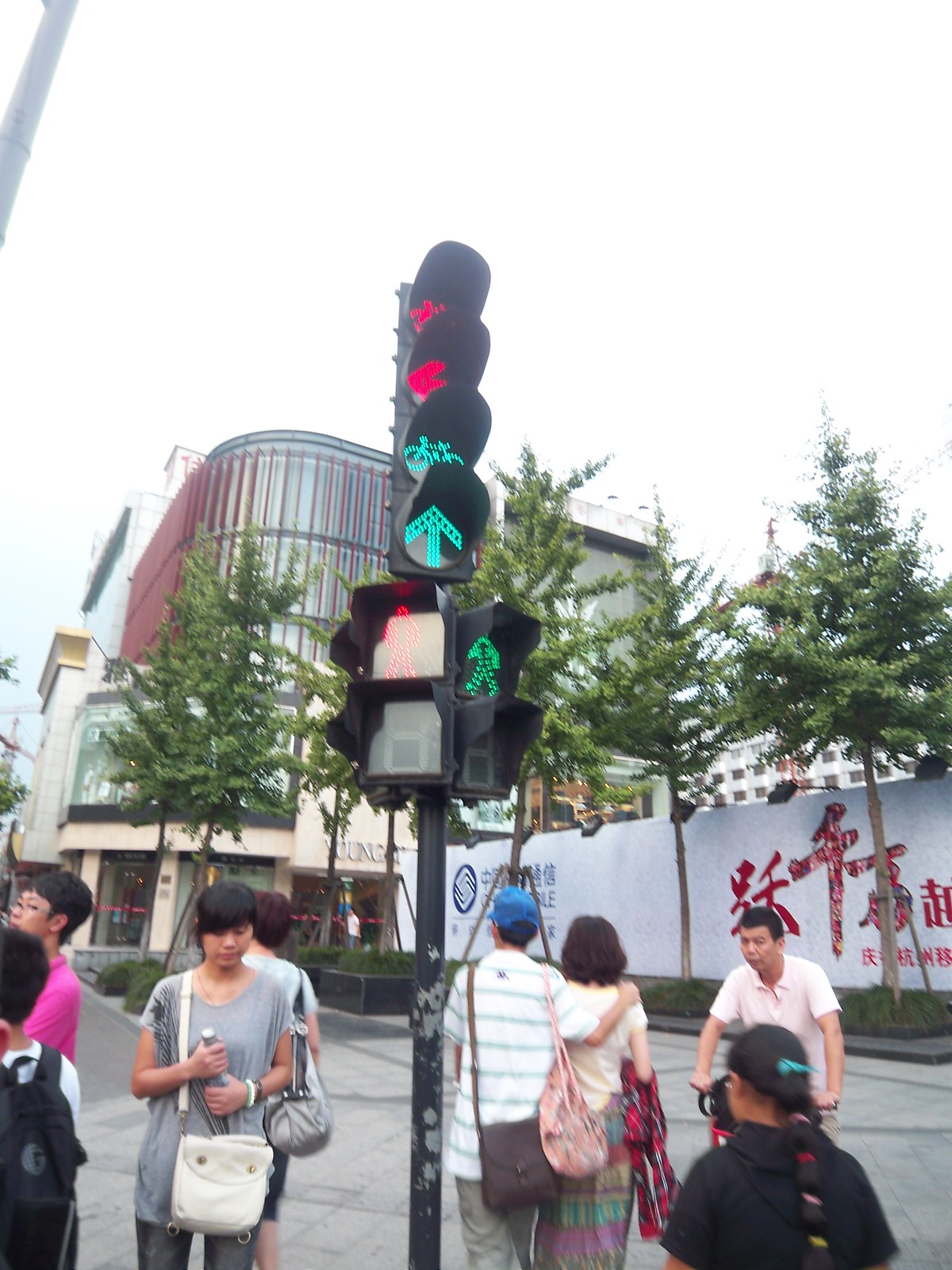The photograph captures a bustling city street in an Asian country, showcasing a diverse group of people either walking or waiting to cross. In the foreground, there's a complex traffic light post featuring multiple signals, including a green arrow, green bicycle, red man, and green man, which add a layer of confusion to the scene. Prominently displayed is a young woman in a gray top holding a white purse, facing towards the camera, complemented by a man in a white and striped polo with a blue hat and tan pants, gently placing his hand on a woman in a white top and multi-striped skirt. The background reveals a modern building with a blue glass facade and curved corners, amidst a scattering of straight-trunked trees that resemble pines from a certain height. Additionally, there is a white wall embellished with red and blue lettering. The wide sidewalk and absence of cars emphasize the pedestrian nature of the area, lending a vivid snapshot of daily urban life in this foreign locale.